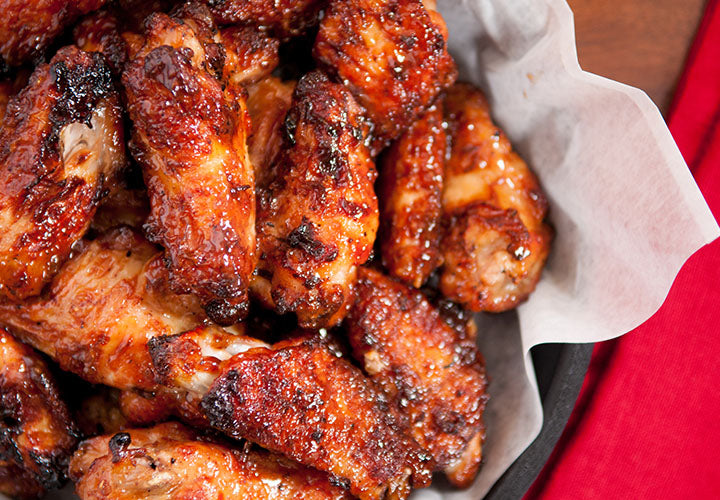The image captures a tantalizing display of chicken wings, neatly arranged in a black basket or dish, lined with a white napkin or towel. The dish is brimming with at least two dozen grilled or baked chicken wings, generously coated in a sauce that gives them a moist and glossy appearance. The wings are stacked high, showcasing a range of textures from charred black points to reddish-brown finishes, with hints of the tender white meat beneath. The setting appears to be on a light brown wooden table, with a red napkin or cloth situated to the right of the basket, adding a pop of color to the scene. The composition, possibly an enticing food advertisement, highlights the wings' rich and savory allure, inviting viewers to savor their enticing aroma and flavor.